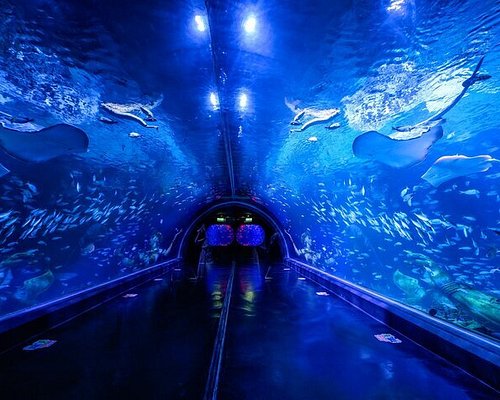The image captures a vibrant scene inside an aquarium tunnel, where visitors can walk through and observe marine life all around them. On both the left and right sides of the tunnel, large glass panels provide a clear view into the aquarium, showcasing a variety of ocean creatures swimming freely. The water is a luminous blue, illuminated by fluorescent white lights above, which create reflections and a serene ambiance. Schools of silver and white fish float gracefully, with larger marine animals such as a white frog and possibly a shark, visible towards the top. The tunnel itself is shaded in black, creating a striking contrast with the bright blue water. At the end of the tunnel, an entrance or exit is noticeable, framed by a couple of windows offering different viewpoints into the aquarium. The photograph emphasizes the immersive experience provided by the tunnel, where both large and small sea life can be observed in their fluid movements on all sides, enveloping visitors in an underwater world.